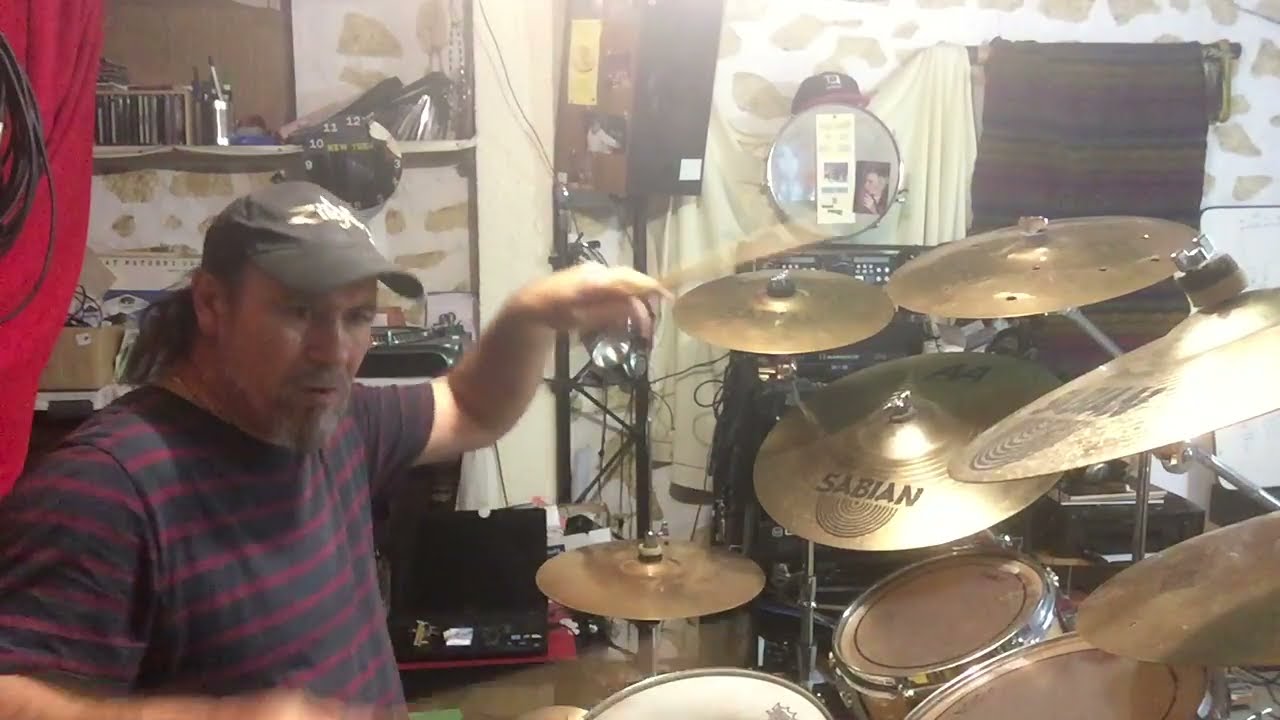The photograph captures an indoor scene with a white-painted wall featuring brown blotches and stripes meant to simulate a brickwork pattern, which resembles a spotted cow. On the left side of the image, a red curtain, intricately looped with black wire, extends almost the full height of the frame. In the foreground, a man with lighter skin, graying beard, and shoulder-length, swept-back gray hair, is sitting and facing right. He is wearing a black ball cap with some unclear golden red writing, and a short-sleeved, red and navy-blue striped shirt along with a gold chain around his neck. His mid-chest to upper body is visible, and his arms are raised as he holds blurred, rapidly moving drumsticks. On the right side of the image, a drum set is prominently featured, including a high-top cymbal, at least five flat cymbals labeled "Sabian," two tom drums, and a snare drum. Additional musical equipment and a small black clock can be seen in the background.